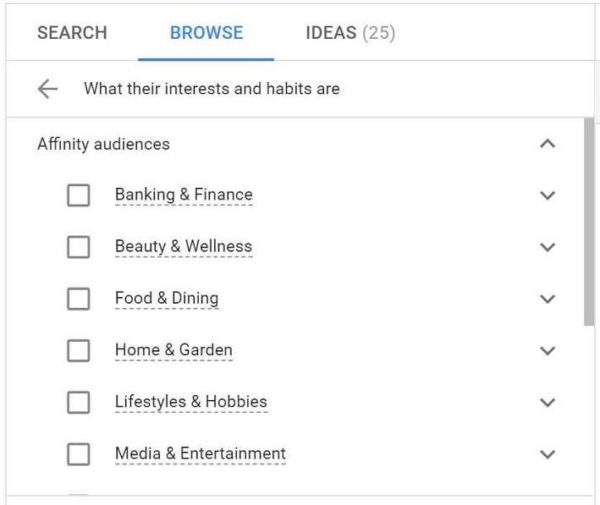The image features a sleek user interface with a predominantly white background. In the upper left corner, the word "Search" is displayed, followed by "Browse" in blue with an underline. To the right, "Ideas (25)" appears in black text. The "Browse" text stands out with its blue color. Below this, a horizontal line separates these elements from the rest of the content. 

Directly underneath, a left arrow is displayed adjacent to the text "Interests and Habits," which is followed by another line of separation. The next section is titled "Affinity Audiences," each item in this list is accompanied by a checkbox on the left and a dropdown menu on the right. The dropdown menu for "Affinity Audiences" is shown as open, revealing a more detailed list underneath.

The detailed list includes categories such as "Banking and Finance," "Beauty and Wellness," "Food and Dining," "Home and Garden," "Lifestyles and Hobbies," and "Media and Entertainment." These items are displayed in a slate gray font against a light gray box, giving a clean and organized appearance.

On the right side of the interface, a scrollbar is visible, indicating that the list can be scrolled to reveal additional categories that are currently not visible in the image. The overall color scheme consists of white, gray, blue, and slate gray, contributing to the minimalist and professional design.

Each interactive element, from categories to dropdown menus, is carefully boxed within light gray borders, enhancing readability and ease of use.